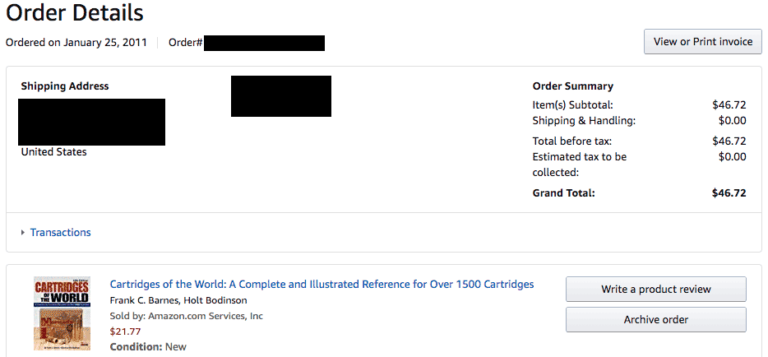This screenshot captures the detailed order summary of a purchase made on January 25th, 2011. In the top left corner, bold black text reads, "Order Details," followed by the smaller text, "Ordered on January 25th, 2011." A small grey vertical line separates this information from the "Order Number," which is blacked out for privacy. On the right side, a grey box with the text "View or Print Invoice" is displayed.

Below this section, there's a large box outlined in grey, containing the shipping address, which is bolded and subsequently blacked out, with "United States" visible underneath. Adjacent to this, another blacked-out rectangle obscures additional information.

Further to the right, another section headed "Order Summary" in bold contains the following details:
- Items subtotal: $46.72
- Shipping and handling: $0.00
- Total before tax: $46.72
- Estimated tax to be collected: $0.00
- Grand total (in bold): $46.72

A grey line and blue text indicating "star" transactions conclude this section.

The screenshot also shows another grey-outlined box featuring the product details. It begins with:
- "Cartridges of the World" written in bold, and an image of a magazine cover titled "Cartridges of the World," with "Cartridges" in red and "of the World" in black text. Below this, a blue bar and an indistinguishable image are seen, all set against a wooden floor backdrop.

Beneath the image, blue text reads: "Cartridges of the World: A Complete and Illustrated Reference for Over 1500 Cartridges." The authors are listed as Frank C. Barnes and Holt Bodenson. The product is sold by "Amazon.com Services, Inc." and priced in red at $21.77. The condition of the product is stated as "New" in bold black text.

To the right of the product details, there is a grey box inviting the customer to "Write a Product Review," with "Archive Order" text below this box.